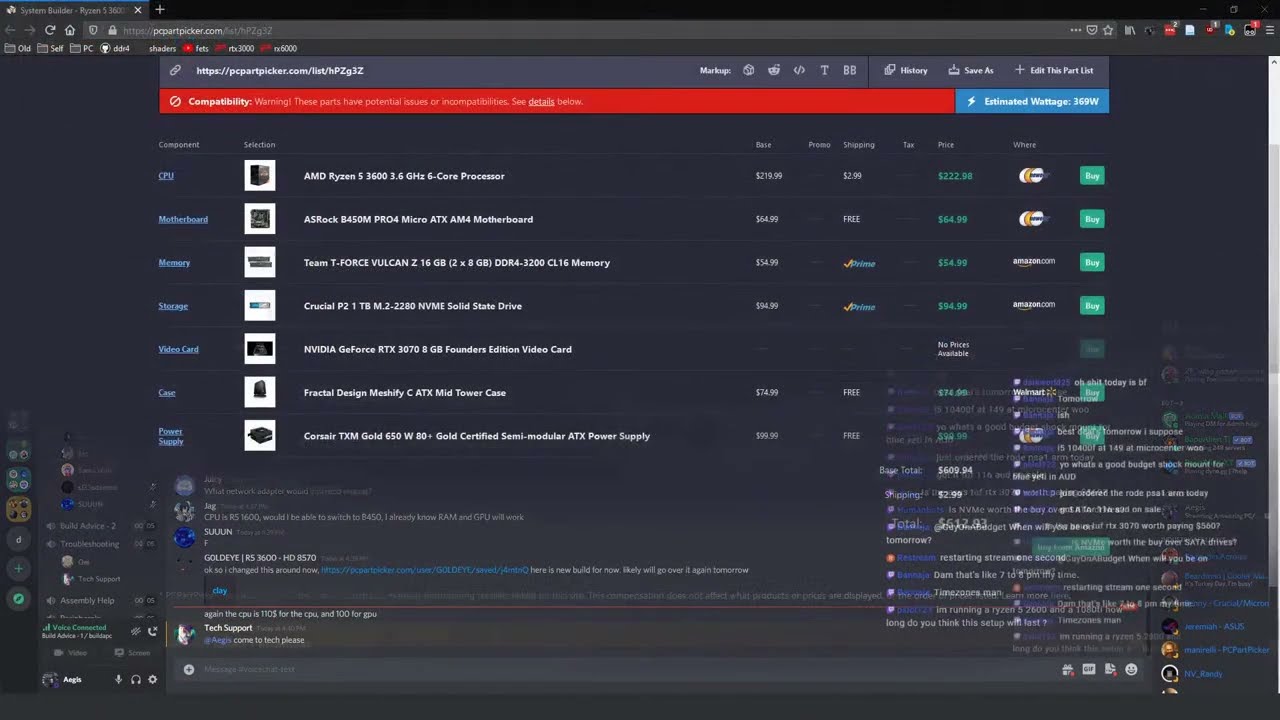The image is a detailed screenshot of a dark gray-themed Discord interface, showcasing an active text channel intended as a supplementary communication method for those in voice chat. The central part of the image is dominated by a chat window filled with lines of text from various users, each accompanied by circular avatars on the left. Though the text is too compressed to be legible, the conversation appears lively and ongoing. On the far left side of the screen, there's a vertical toolbar featuring several icons, including the Discord logo, a power symbol, and an icon for the video game Overwatch, along with application folders. Adjacent to this toolbar is a channel list displaying different available chat rooms. On the far right, there's a friends list panel showing users' statuses, such as online or offline. The overall image is organized into multiple panes and tabs with a consistent layout of white and blue text contrasted against the dark background, punctuated by colorful user icons and various menu options.